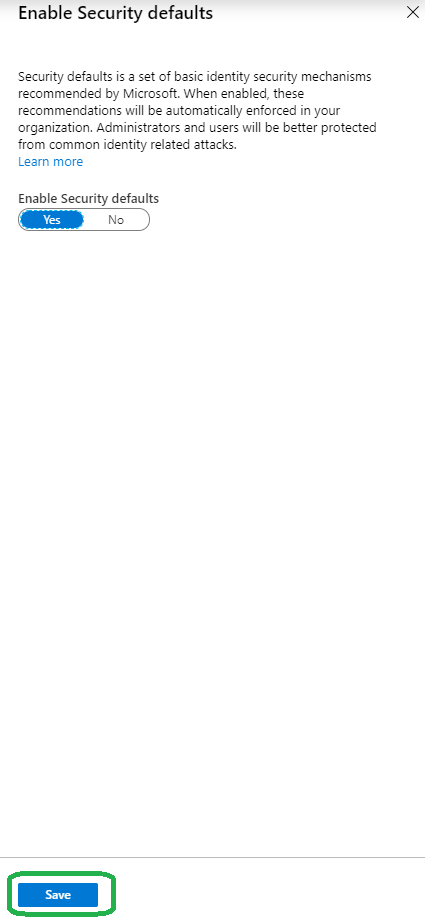A screenshot displays the "Enable Security Defaults" settings page within a Microsoft administrative interface. In the top right corner, there is an 'X' for closing the window. The page includes a description that reads, "Security Defaults is a set of basic identity security mechanisms recommended by Microsoft. When enabled, these recommendations will be automatically enforced in your organization. Administrators and users will be better protected from common identity-related attacks." 

Below this description, there is a clickable "Learn More" link highlighted in blue. Beneath the link, a section labeled "Enable Security Defaults" presents a horizontal toggle option with "Yes" on the left side and "No" on the right side. The "Yes" option is selected and highlighted in blue, indicating the current choice for enabling Security Defaults.

At the bottom of the screenshot, there is a "Save" button, also highlighted in blue and surrounded by a green border, indicating that it is ready to be clicked to save the current settings. This screenshot illustrates the precise steps within the interface where an administrator can enable Security Defaults to enhance the security measures for their organization.